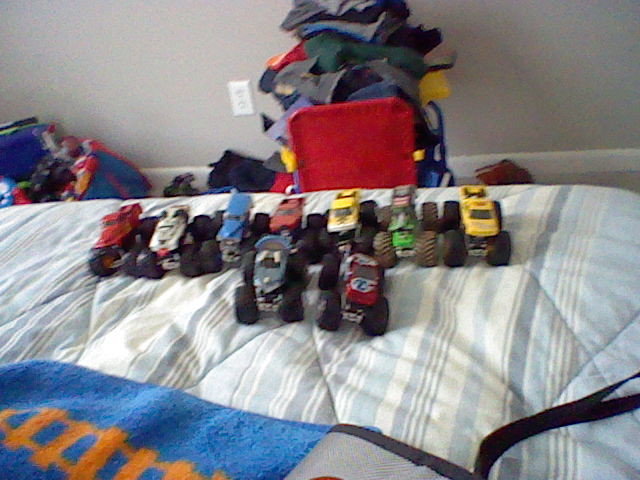This is a color photograph depicting a collection of toy monster trucks meticulously arranged on a bed or couch. The vehicles are aligned in two rows: a longer one in the back and a shorter row of two in the front. Each truck, characterized by large, dark wheels and vibrant bodies, comes in various shades including red, blue, yellow, and green. They are set against a quilted cover adorned with blue and white vertical stripes, which appear somewhat crumpled. 

In the foreground, to the left, lies a plush blue object with an orange ladder printed on it. Also notable is a small grey object with white outlines positioned at the bottom center. The background features a red box brimming with clothes and fabric items, next to another smaller but equally overflowing box in the upper left corner. The surrounding floor area has indistinguishable items scattered across it. The backdrop consists of a light grey wall accented with a cream or white skirting board, and beneath that, grey flooring. A white power socket is visible just to the left of the large box filled with clothes.